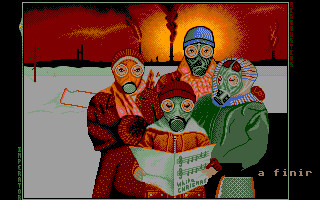A vivid and haunting colored sketch or painting of a four-member family—comprising a mother, a father, and two children—depicts them all wearing gas masks amidst a dystopian backdrop. The family is dressed in winter attire, suggesting a harsh and cold environment. In the background, towering factories and the ominous glow of a nuclear explosion or bomb blast dominate the scene, while snow gently falls, adding to the eerie atmosphere.

The father stands at the back, wearing a blue beanie, a green gas mask, and a scarf snugly wrapped around his neck. To his right stands the mother, who is donning a red polka dot coat, coupled with an orange scarf, an orange gas mask, and a striped red beanie. The youngest child, likely a boy, is situated in front of his mother. He is attired in a brown jacket with a wool hoodie, a red beanie, and a green gas mask. Clutching a musical book titled "White Christmas," adorned with music notes, he adds a poignant contrast to the bleak surroundings. The sister or daughter stands to the right, wearing a green jacket and gas mask, her face obscured but her presence adding to the family's stoic unity in the face of adversity.

The detailed winter clothing, the chilling nuclear backdrop, and the juxtaposition of traditional festive symbols with survival gear create a powerful and thought-provoking image.